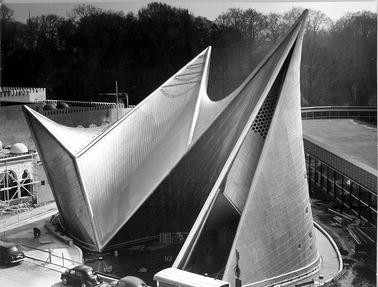This black-and-white photo captures a striking outdoor scene featuring an architecturally unique building. The building, tall and prominent, has three distinct pointy tips and incorporates a spiral-like structure on its backside, resembling an 'S' shape. Silhouetted against a light gray skyline, the sun appears to be setting, casting a gentle glow over the trees on the right side, making them appear lighter compared to the darker, silhouette-like trees on the left. Surrounding the focal building are smaller structures and parked cars, emphasizing the building's towering presence. In the background, a dense treeline, possibly a forest, adds depth and context to the scene, combining natural and man-made elements harmoniously.